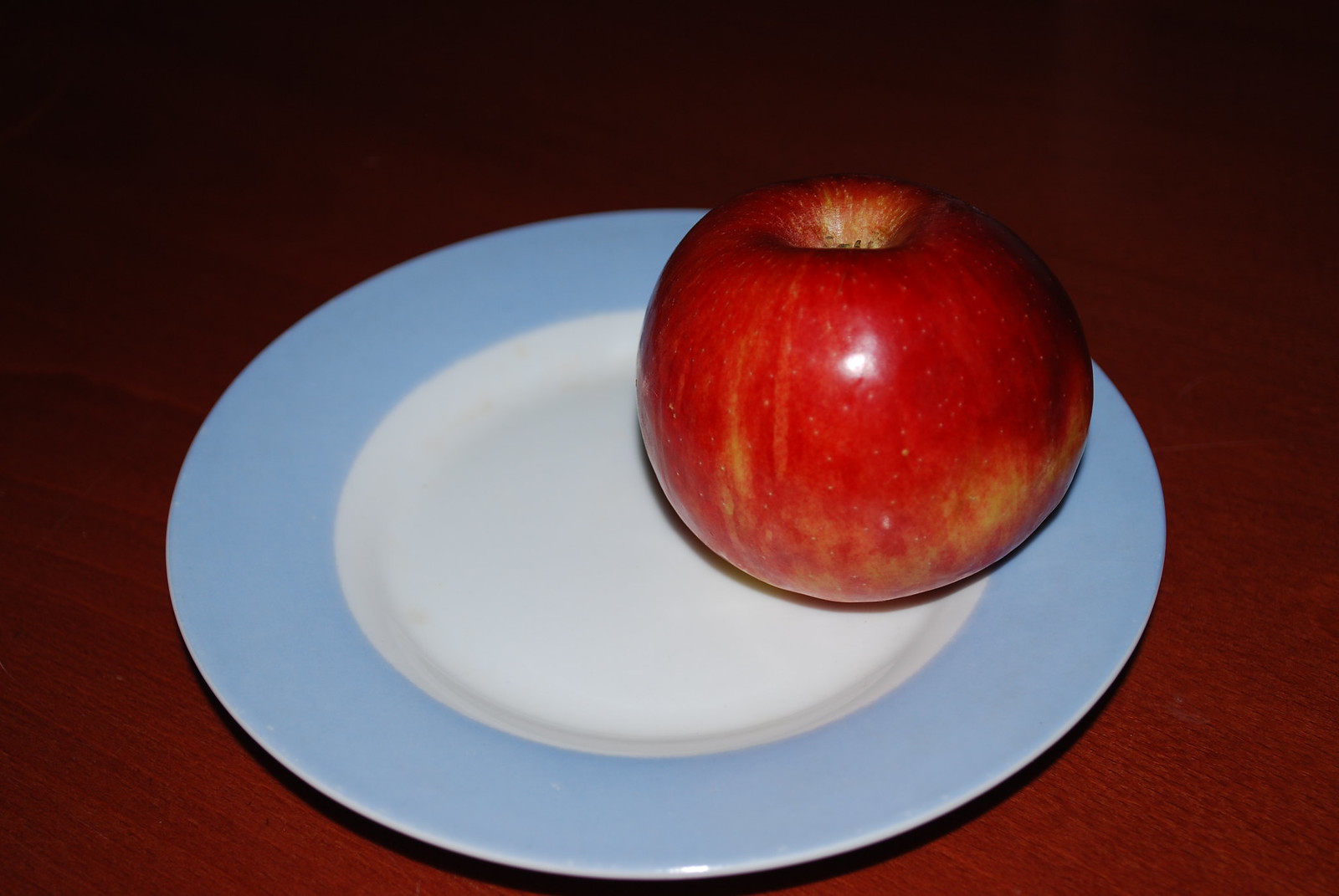A beautifully crafted table made of rich, reddish-brown wood occupies the foreground. The dark upper part of the image obscures the table's surroundings, drawing attention to the exquisite wood grain. On the table rests a small, light blue-rimmed plate with a pristine white center. Placed on the right side of the plate is a single, vibrant red apple, shining with reflected light. The apple, positioned upside down, reveals its slightly yellow and russet-colored bottom. The front of the apple features subtle yellow streaks, adding to its striking appearance. There is a delicate shadow cast towards the upper right of the apple, enhancing its glossy texture and three-dimensional form.